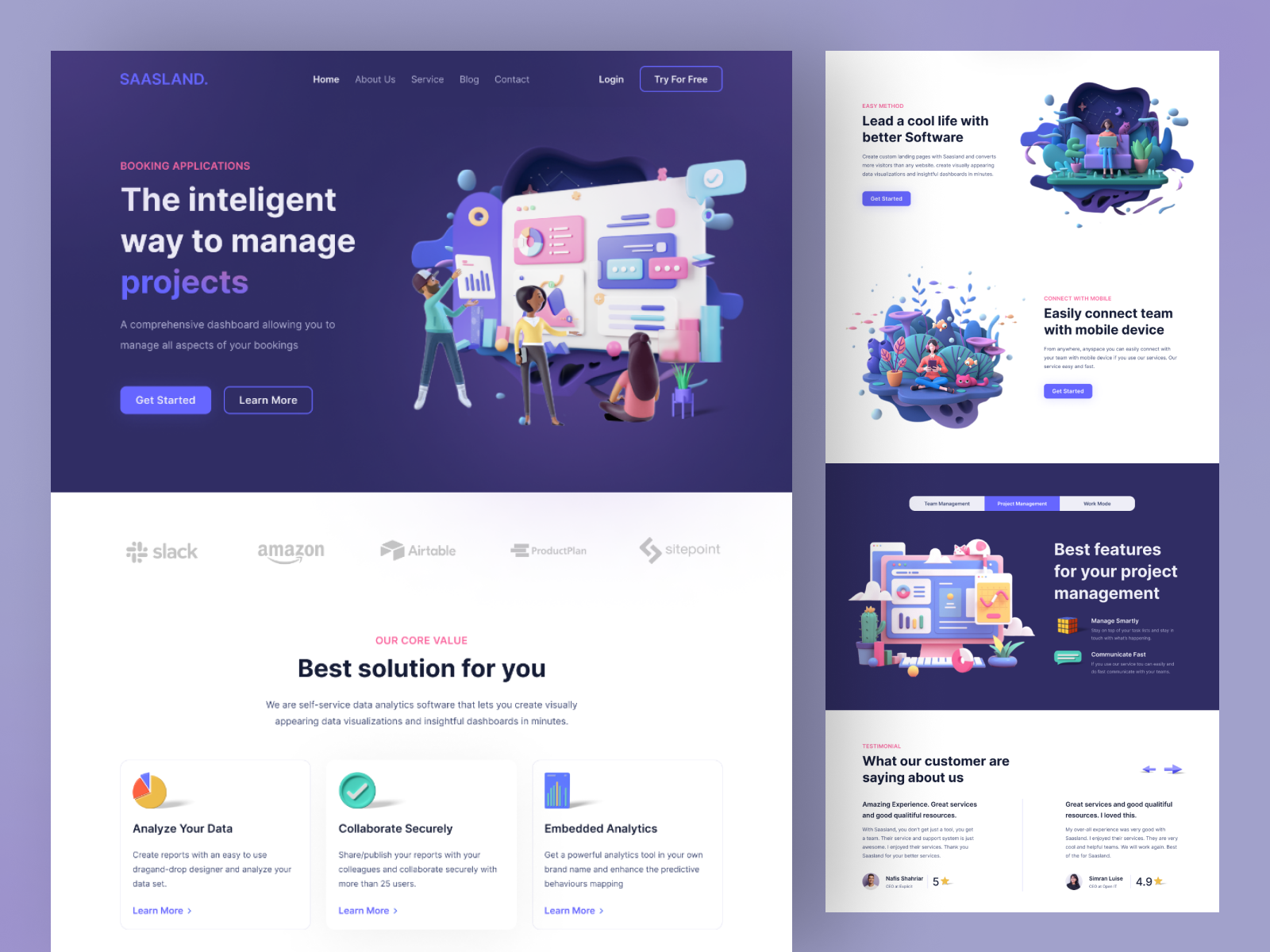The top left corner of this webpage features a navy blue rectangle with the text "SAAS LAND" in blue. Just to the right are the options to "Log In" and "Try for Free." Below that, on the left side, is a light gray rectangle with another navy blue rectangle inside it containing "SAAS LAND." Below this, the text "Booking Application" is prominently displayed in red, followed by "The intelligent way to manage" in white, "Projects" in blue, and the options "Get Started" and "Learn More" also in blue.

On the right side of this area, there is an image resembling a billboard displaying a webpage. In front of this billboard is a little girl sitting with her animal, alongside her mother and father, all gazing at the billboard.

Beneath the blue rectangle, a white rectangle contains text proclaiming "Best solution for you." Further down, it lists features like "Analyze your data," "Collaborate securely," "Embedded analytics." Adjacent to this, on the right, a white triangle reads "Lead a cool life with better software" and depicts the same family engaging in various activities: sitting on a couch with a laptop, the mother or daughter sitting outside with plants and a cat. The section emphasizes "Easy connection and team collaboration with mobile devices" and shows a computer screen displaying different websites with the caption "Best features for your project management."

At the bottom of the page, a white rectangle hosts testimonials saying "What our customers are saying about us." It contains small-print paragraphs on the left and right sharing different customer experiences.